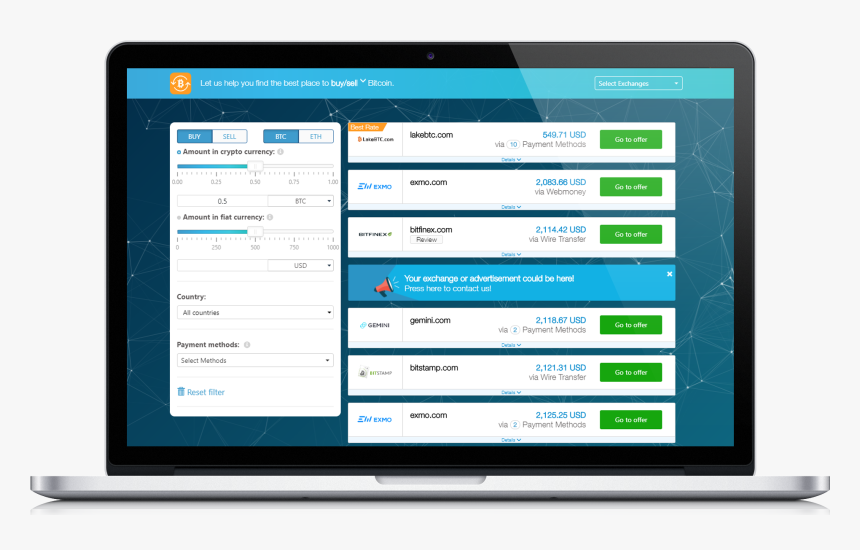The image showcases an open laptop with a silver-gray base and a screen framed in black. Displayed on the screen is a website dedicated to facilitating Bitcoin transactions. At the top of the website, a light blue bar prominently features the text: "Let us help you find the best place to buy/sell Bitcoin." To the right of this bar is a dropdown menu labeled "Select exchanges."

The main interface of the website is set against a blue background adorned with constellations. A navigation tab on the left side allows users to switch between "Buy" and "Sell" modes, with the "Buy" and "ETC" options currently highlighted. Below, in bold text, are two sliders for transaction amounts: "Amount in Cryptocurrency," which ranges from $0 to $1 and currently set at 50 cents, and "Amount in Fiat Currency," extending from $0 to $1,000 and set at $500 USD. Additional dropdown menus allow the selection of the country (with "All countries" as an option) and payment methods (with "Select methods" dropdown).

On the right side of the screen are several rectangular boxes showcasing different exchanges and their corresponding offers. Each box includes a logo, the exchange's name, price in USD, and a "Go to offer" button. The exchanges listed are:
1. lakebtc.com at $549.71 USD.
2. exmc.com at $2,083.66 USD.
3. bidiflix.com at $2,114.42 USD.

An advertisement interrupts the list with a blue banner reading: "Your exchange, Our advertisement could be here. Press here to contact us," accompanied by a speakerphone illustration.

Continuing below the ad, additional exchanges are listed:
4. gemini.com at $2,118.67 USD.
5. bidstep.com at $2,121.31 USD.
6. exmc.com at $2,125.25 USD.

Each exchange listing also indicates the acceptable payment methods in gray text beneath the price.